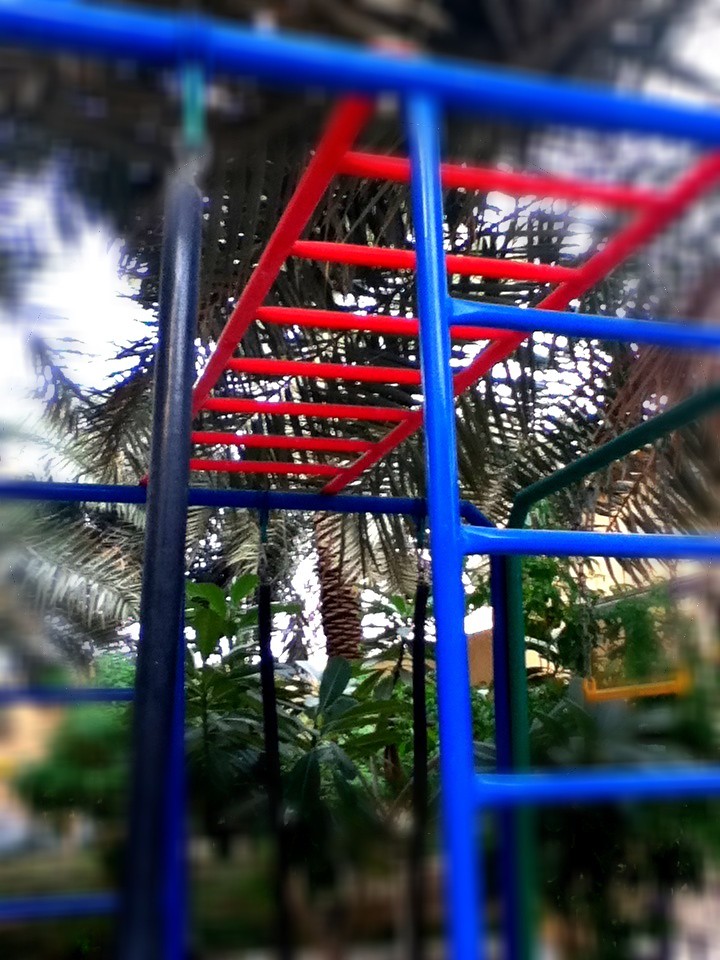The image depicts a vibrant playground structure in red and blue, set against a tropical backdrop. In the foreground, there's a dark blue vertical ladder leading up to a horizontal red bar that spans across the top of the frame, serving as an overhead climbing apparatus. The upper section features a side-on red ladder with connecting bars, creating a network for children to traverse hand-over-hand. Closer inspection reveals various shades of blue bars—dark blue on the left and light blue on the right—that form intricate connections, some extending beyond the image. The right side of the playground is clearer, showcasing the prominence of the red ladder. 

Surrounding the playground, palm trees are visible both in the background and foreground, with some green palms near the base of the structure. A hint of a cloudy sky frames the scene, adding depth. In the distance, on the right side, there is a yellow building, possibly a school, faintly visible. The left side of the image is slightly blurry, contrasting with the sharp focus on the playground's right side and its red upper ladder. This detailed playground photograph captures the essence of a lively, tropical environment.